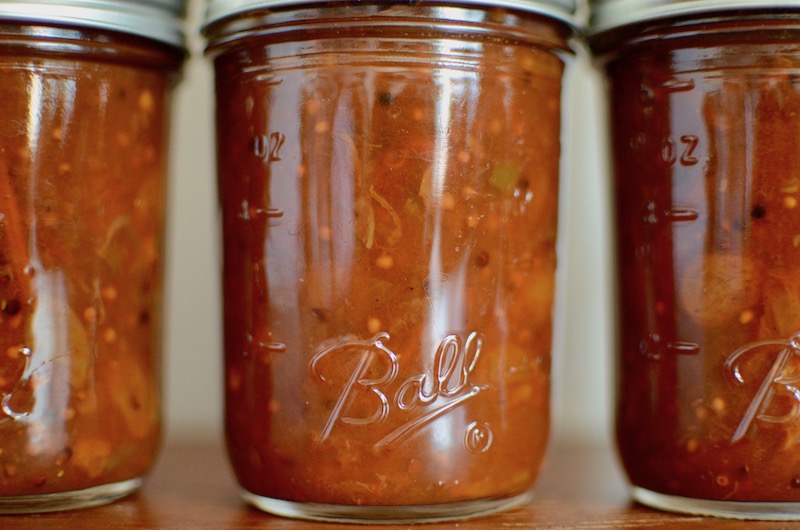This detailed, artistic close-up image features three identical, transparent glass jars prominently displayed on a wooden surface. The jars are filled with a rich, red substance that resembles homemade tomato sauce or a tomato-based stew, suggesting an organic and preserved culinary creation. Each jar is embossed with a raised, cursive "Ball" logo, complete with a registered trademark symbol at the bottom right. These Ball mason jars also feature gradations and measurement markings along their sides, with visible increments at 2, 4, and 6 ounces. The jars have white, screw-on lids, though they might appear metallic from certain angles. The setup is enhanced by natural lighting, giving the image an inviting, bright, and clear appearance. The central jar is fully visible, while the jars on either side are partially obscured, creating a balanced, aesthetically pleasing composition that highlights the artisanal nature of the preserved contents.